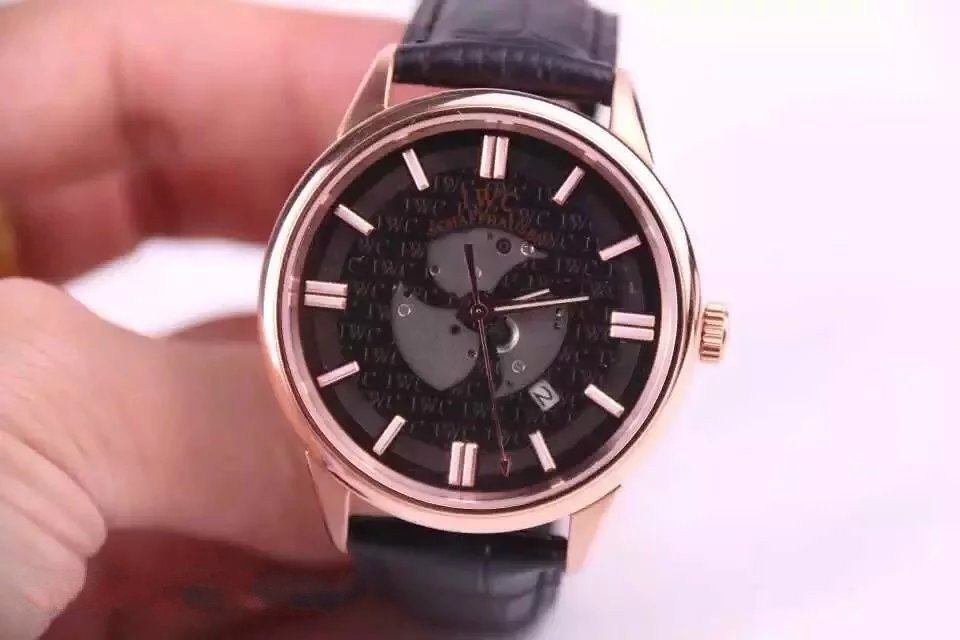In this close-up photograph of a watch face, a white hand holds the timepiece, with the left pointer finger distinctly visible. The watch, which appears to be a men's model, has a slight pink hue in the image that may suggest an anomaly in the photo's coloring, possibly disguising its true silver metal finish. Both top and bottom holders are attached to a black leather band. The watch face features unique numerical indicators: the 1 and 2 are marked with single lines, while the 3 and 6 have two lines. This pattern continues around the dial up to 12. The hour and minute hands display a time of approximately 2:14, and there's a longer second hand pointing to around 27 seconds, which may be red. The background of the clock face is a lighter gray, showcasing some visible inner mechanisms and scattered, unreadable letters. A large and prominent number "2" is also evident within the design.